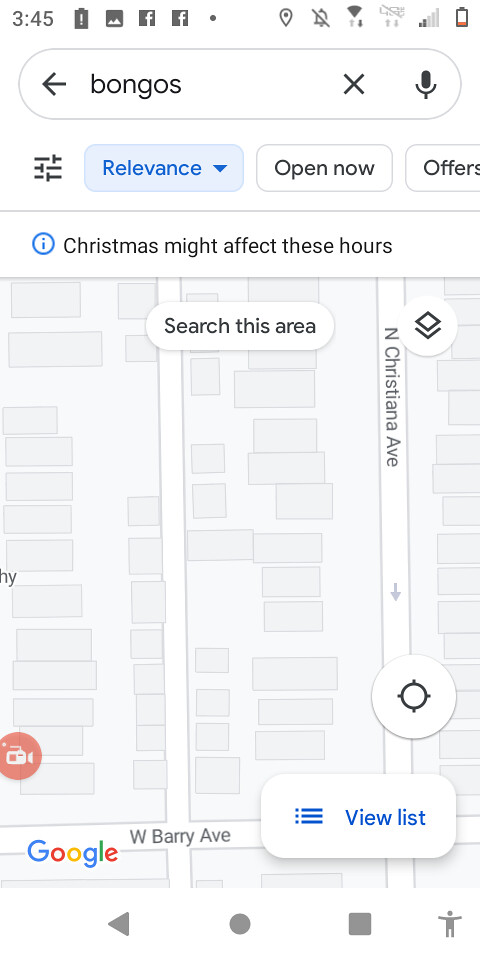The screenshot captures an Android smartphone displaying the Google Maps app. At the bottom, the distinct Android navigation icons—back button, home circle, and recent apps square—confirm the device's operating system. The status bar at the top shows the time as 3:45, along with several notifications: one for low battery, one for photos, and two from Facebook. Active icons include location services, a muted bell indicating silent mode, a Wi-Fi symbol with alternating arrows (presumably indicating data transfer), and a cellular signal with two filled bars. The upper right corner prominently features the low battery indicator.

Focusing on the main content, the Google Maps app is open with "bongos" entered in the search bar. The map beneath is zoomed into a neighborhood view, showing a grid of streets and structures. It does not display the Street View mode, but rather a standard map layout with clearly defined rectangular plots representing buildings and lots. This detailed setup captures a typical usage scenario of an Android phone user searching for a specific location on Google Maps.